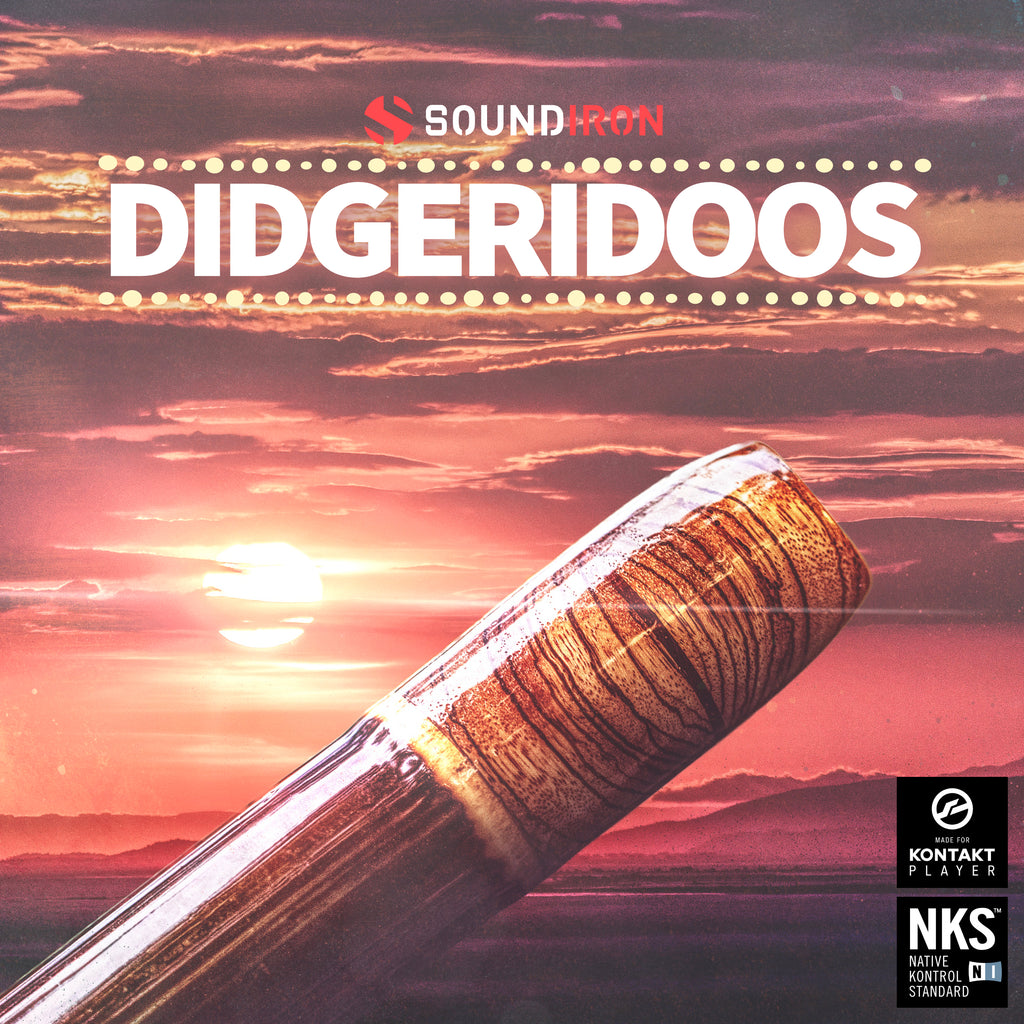The image, which appears to be a cover possibly for an album or a product, is square-shaped, measuring approximately five to six inches on each side. The background is a sunset scene dominated by a vibrant sky with streaks of clouds, primarily orange, with hues of reddish-purple. This sky occupies the upper three-fourths of the image, while the lower section features some indistinct low-lying hills or a valley.

In the lower left corner, a bright white sun emits an orange glow, casting a warm tone over the scene. At the top center of the image, there’s a small, red circle logo with two lines taken out of it, and next to it, the word 'Sound' appears in white text, followed by 'Iron' in red text, combining to spell 'Soundiron.'

Below this logo, the word 'Didgeridoos' stands out in bold, large, white print, spreading across the width of the image. This text is flanked by two horizontal rows of small yellow circles. The focal point of the image, a long, highly-polished wooden didgeridoo, extends diagonally from the lower left corner towards the center-right.

In the lower right corner are two black squares stacked vertically, with white text. The top square reads 'Made for Kontakt Player,' and the bottom square reads 'NKS, Native Kontrol Standard.'